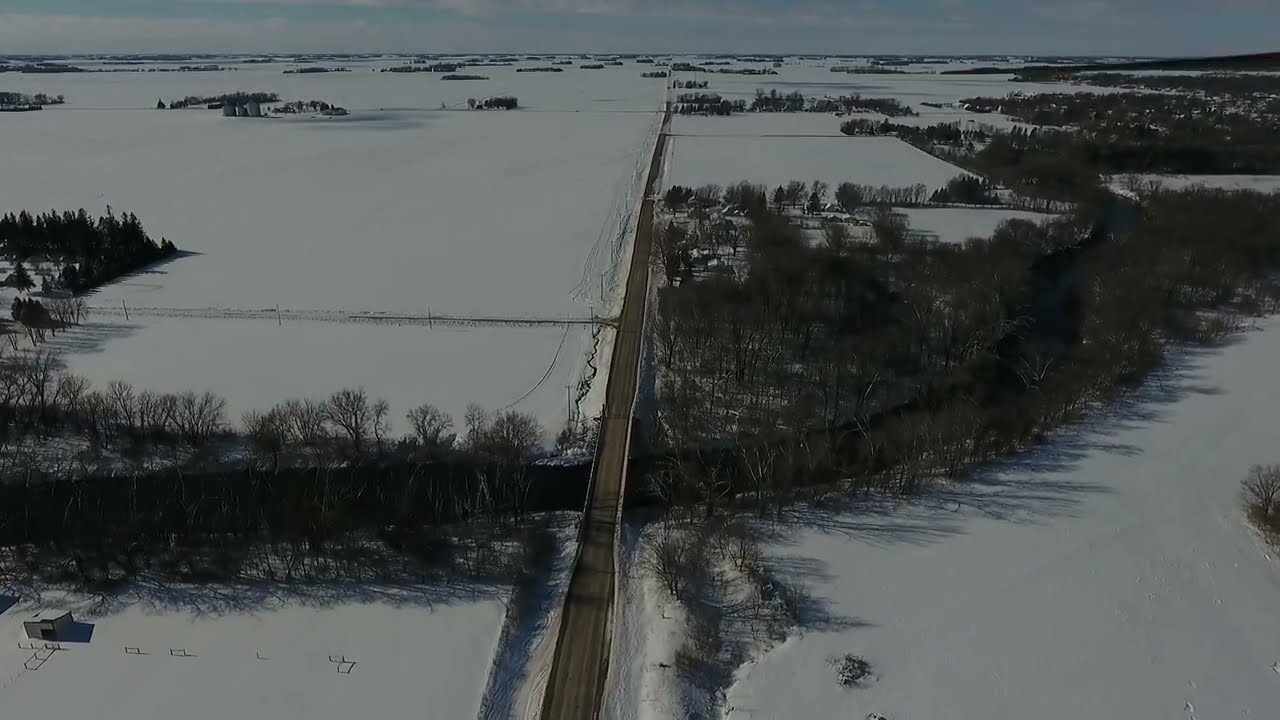This aerial drone photograph vividly captures a wintry landscape featuring a central, dark gray road. The road stretches from the foreground, narrowing as it recedes into the distance towards the top center of the image. Flanking this road are expanses of pristine, snow-covered fields, occasionally disrupted by tire marks, especially on the left side of the image, while the right side remains untouched and smooth.

A notable feature in the foreground is a bridge spanning a river or stream, oriented horizontally from left to right across the image. The bridge reflects the same clear, dry pavement as the main road, contrasting sharply with the surrounding white snow. Dotting the borders of these snowy fields are rows of barren, brown trees, stripped of their foliage.

An electricity wiring tower or radio tower is also visible on the right side of the image, adding a touch of industrial presence to this tranquil scene. Overhead, the sky is a pale to medium blue, decorated with light, fluffy clouds, completing this picturesque, serene snapshot of a winter day.